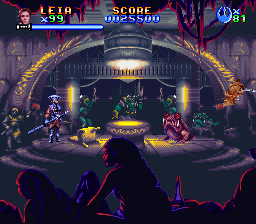This image is a screenshot from a video game, depicting an intense battle scene set on a dark brown stage. The stage is centered around a dark gray cauldron filled with an orange, glowing liquid that seeps out. Two main characters are engaged in combat: one is adorned in purple armor with matching purple boots over a dark brown undercoat, while the other is cloaked in a dark black robe, has dark skin, and black hair. In the background, green, alien-like monsters with golden hair and red eyes add to the chaos, along with a golden statue situated to the left. The scene is illuminated by a cylindrical light above, casting shadows and a mix of purple and red hues upon the audience, who are rendered in dark tones.

On the left side of the image, there’s an overlay of a man's face with short, round hair and light skin. Next to this face, in orange text with yellow highlights, it reads "LEIA," followed by "X99" where the 'X' is in blue and the '99' in lime green. In the upper right corner, an icon resembling a tree inside a circle with the text "81" is visible; the tree and ‘X’ are blue, while the '81' is lime green. Across the center of the screen, the word "SCORE" appears in bold orange text with a yellow outline, beneath which a score of "0025500" is displayed in dark blue with a lighter blue stripe running through it. The overall setting gives the impression of an arena or cavern, with archways and spikes, adding an extra layer of depth and intensity to the scenario.